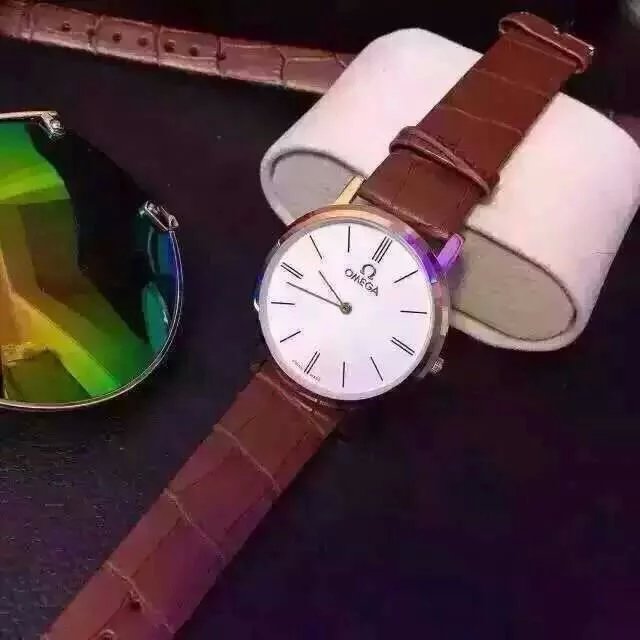This image appears to be an advertisement showcasing an Omega analog watch with a distinct vintage aesthetic. The prominent watch features a classic circular dial framed by an elegant gold trim, adorned with the iconic Omega logo at the center. Roman numerals are intricately displayed around the dial, although they seem to follow an unconventional arrangement. The watch is complemented by a rich brown leather strap that drapes diagonally from the top right to the bottom left of the frame, adding to its sophisticated appeal.

Resting on a pristine white rectangular case, possibly the watch's own presentation box, the setup exudes an air of luxury and refinement. Another brown strap, likely an accompanying accessory, lies subtly behind the case, from the top left toward the center, further enhancing the composition of the scene.

On the left side of the image, a stylish pair of aviator sunglasses with reflective lenses, tinted in shades of green and yellow, adds a touch of modern flair. While these sunglasses serve as a secondary focal point, the Omega watch undeniably remains the star of this meticulously arranged and granulated photograph.